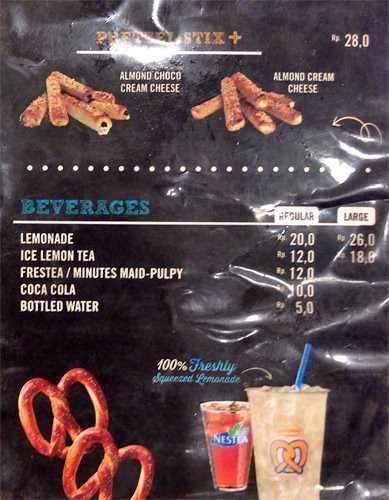The image displays a fast-food restaurant menu with a black background, likely for a pretzel shop, featuring brightly lit text and images. At the top, in yellow and gold letters, it announces "PD Sticks Plus" with a white line underneath. To the top right, "RP28.0" is highlighted. Central to the poster are images and descriptions of various pretzel sticks: "Pretzel Stick," "Almond Choco Cream Cheese," and "Almond Cream Cheese," each accompanied by a picture. A squiggly line and dots separate these pretzel descriptions from the beverage section, which is labeled "Beverages" in blue text with a white line beneath.

The beverage menu lists "Regular" and "Large" sizes (likely priced in rupees, as denoted by 'RP') for the following drinks: Lemonade (RP20.0, RP26.0), Iced Lemon Tea (RP12.0, RP18.0), Freshta/Minute Maid Pulpy (RP12.0), Coca-Cola (RP10.0), and Bottled Water (RP5.0). Descriptions include sizes such as 20, 12, 12, 10, 5, 26, and 18 ounces. At the bottom middle, the text proudly proclaims "100% Freshly Squeezed Lemonade" in white and blue letters, illustrated by a yellow lemonade cup with a blue straw and a pretzel on the glass. Next to it, there's a brown-colored Nestea glass marked with the Nestea logo, and to the left are two typical brown twisted pretzels. The overall appearance of the poster suggests advertisements for a variety of pretzel-based snacks and a range of refreshing beverages offered by the establishment, which might be associated with Auntie Anne’s.